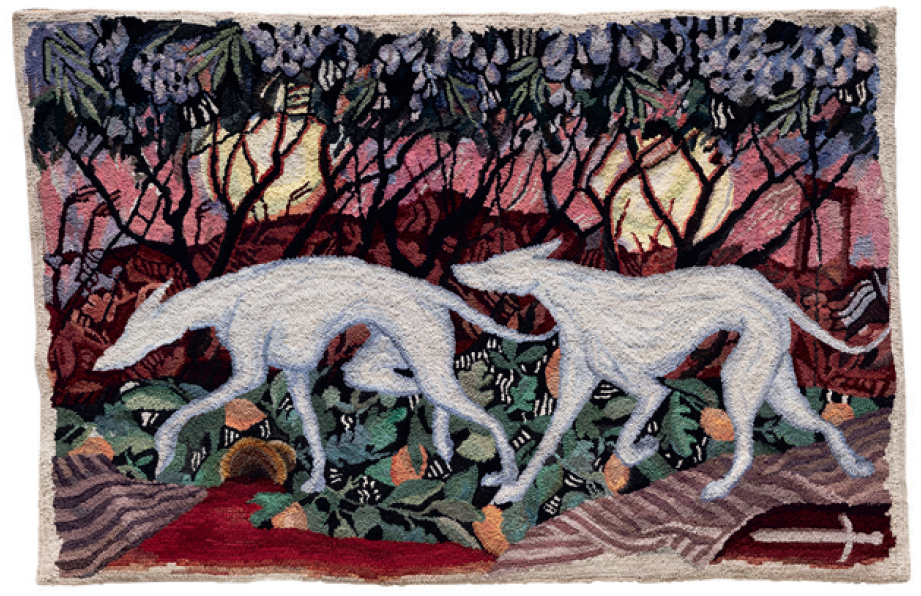This painting features two slender, white silhouettes of canine animals, likely greyhounds or wolves, positioned centrally and walking in single file. The dogs, devoid of any visible details like eyes, appear to be gracefully treading across a landscape that alternates between areas of green, presumably grass, and patches of red. The scene is richly colored, with the background vividly depicting an almost otherworldly environment. Above the dogs, the backdrop includes bursts of pink, light yellow, and red hues, interspersed with dark-trunked trees whose leaves range in color from light blue to lavender. Amongst the foliage, certain plants with green leaves and purple flowers are closely packed together, with stems accented by black and red pin-like details. A prominent feature in the bottom right corner of the painting is a white sword resting on a red surface, resembling a signature. The entire image is bordered by a shade of green, while the overall atmosphere suggests a surreal and colorful woodland setting bathed in unusual light.